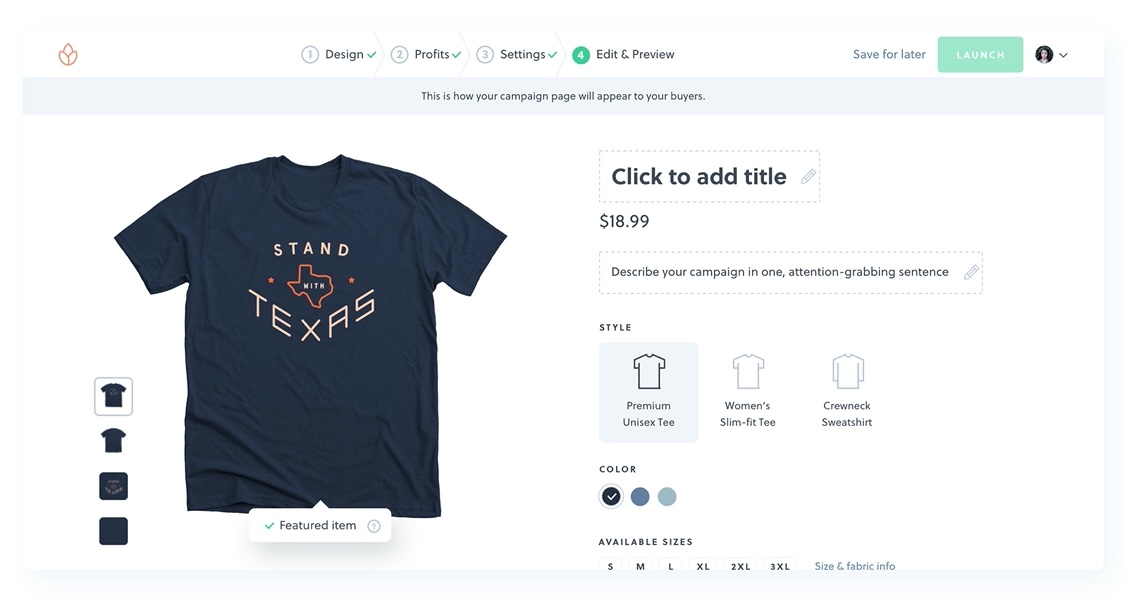This image is a detailed screenshot of a website for purchasing a t-shirt. At the top-left corner, there is an orange minimalist logo resembling a flower, which consists of three ovals. Along the top navigation bar, there are four steps listed: "One Design" (with a green checkmark), "Two Profits" (with a green checkmark), "Three Settings" (with a green checkmark), and "Four Edit and Preview" (highlighted in green). 

On the right side of the top bar, there are options to "Save for Later," a green "Launch" button, and a profile photo inside a circular frame. Directly below the navigation bar, a line of text states, "This is how your campaign page will appear to your buyers."

On the left side of the page, the main product image shows a t-shirt in a dark blue or black color, featuring the text "Stand with Texas." The word "with" is small and situated inside an orange outline of the state of Texas, flanked by two orange stars.

To the right of the product image, there is a placeholder text that says "Click to add title," below which the price "$18.99" is displayed. Following that, there is a space marked, "Describe your campaign in one attention grabbing sentence."

The t-shirt style listed is "Premium Unisex Tee," which is currently selected. Adjacent to that, there are alternate style options: "Women's Slim Fit Tee" and "Crew Neck Sweatshirt." 

Further below, the t-shirt color options available are black, dark blue, and a lighter blue or greenish color. The available sizes are listed as S, M, L, XL, 2XL, and 3XL, with an additional option to click and see the size and fabric information.